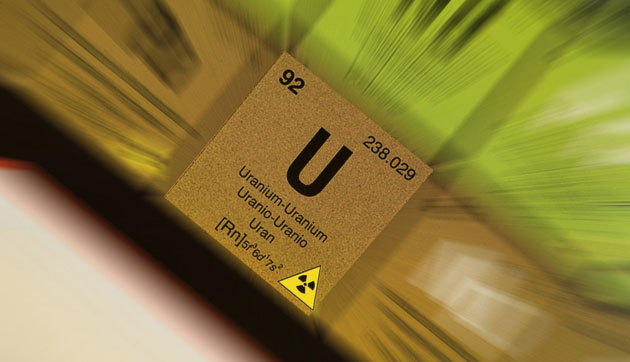In this dynamic and abstract depiction of the periodic table, a central brown tile dramatically highlights the element Uranium, element 92. The surrounding elements are blurred, evoking a hyperdrive effect seen in movies, drawing the viewer’s focus squarely on Uranium. The tile itself is diagonally placed in the center of the image amidst a backdrop featuring bright green vertical lines on the upper right and a solid pink color in the bottom left corner.

The brown tile prominently displays Uranium’s significant details in bold black text: 
- In the upper left corner, "92" signifies the atomic number.
- A large "U," Uranium’s chemical symbol, dominates the center.
- The upper right corner features its atomic mass, "238.029."
- Centered beneath the symbol are the names "Uranium-Uranium" and their translations "Uranio-Uranio," followed by "Uran."

Further details include the electron configuration listed at the bottom of the tile: "Rn 5f^3 6d^1 7s^2," enclosed in brackets. In the lower right-hand corner, a yellow triangle bearing a black biohazard symbol, a striking visual warning of Uranium’s hazardous nature, anchors the design. This vivid depiction effectively underscores the key attributes and danger associated with Uranium.